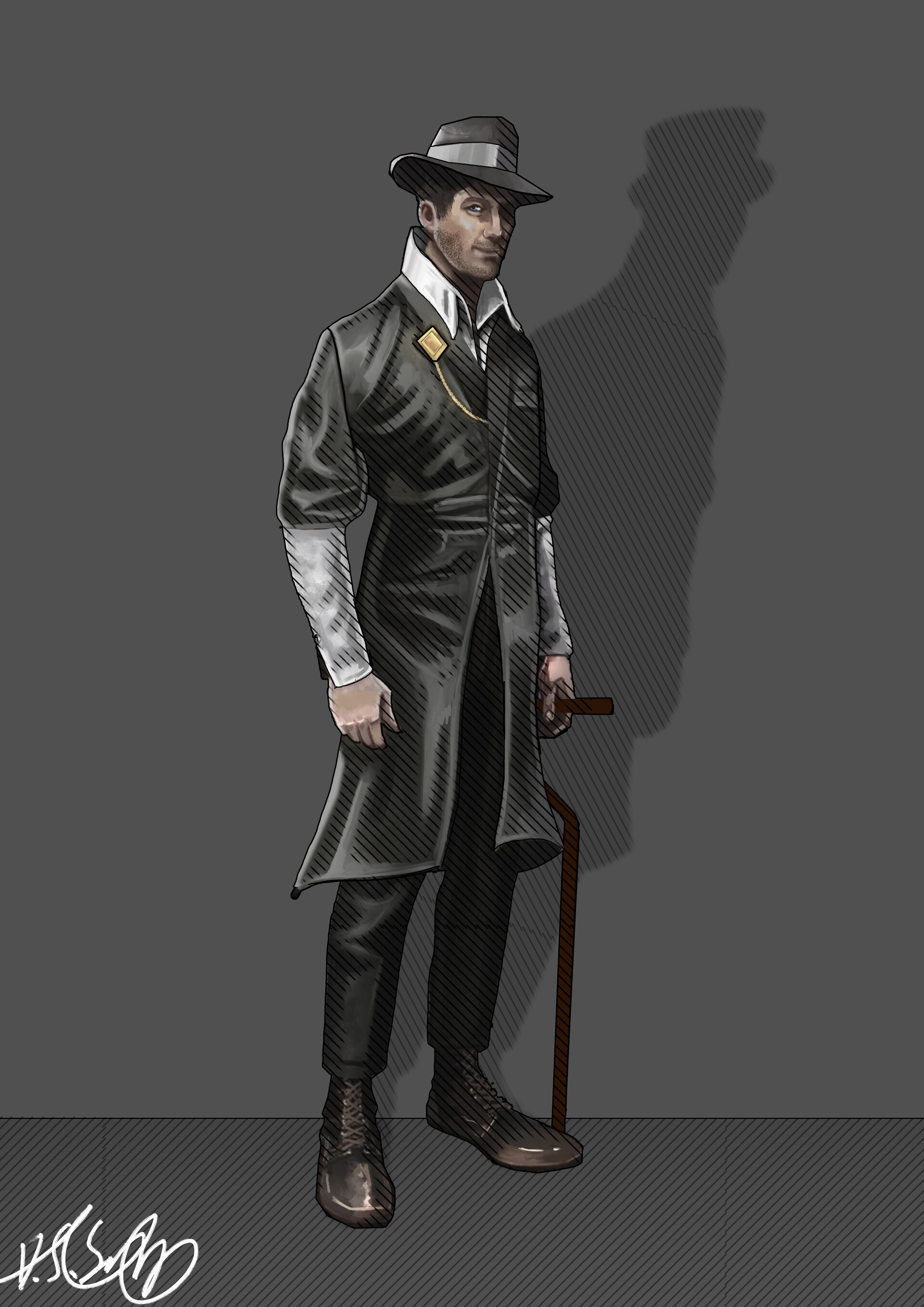This detailed digital illustration depicts a cartoon-style, Caucasian man standing on a darker gray floor with diagonal lines that extend into his shadow. The man, set against a medium gray wall, is attired in a knee-length, short-sleeved black robe with exposed white long sleeves and a tall white collar peeking out. His outfit is completed with black pants, black boots with exaggeratedly large feet, and a dark fedora adorned with a gold brooch pinned to his collar, connected by a chain disappearing inside his coat. He holds a peculiar cane in his right hand and gazes directly at the viewer with one eye. In the bottom left corner, the artist's illegible white signature is visible.